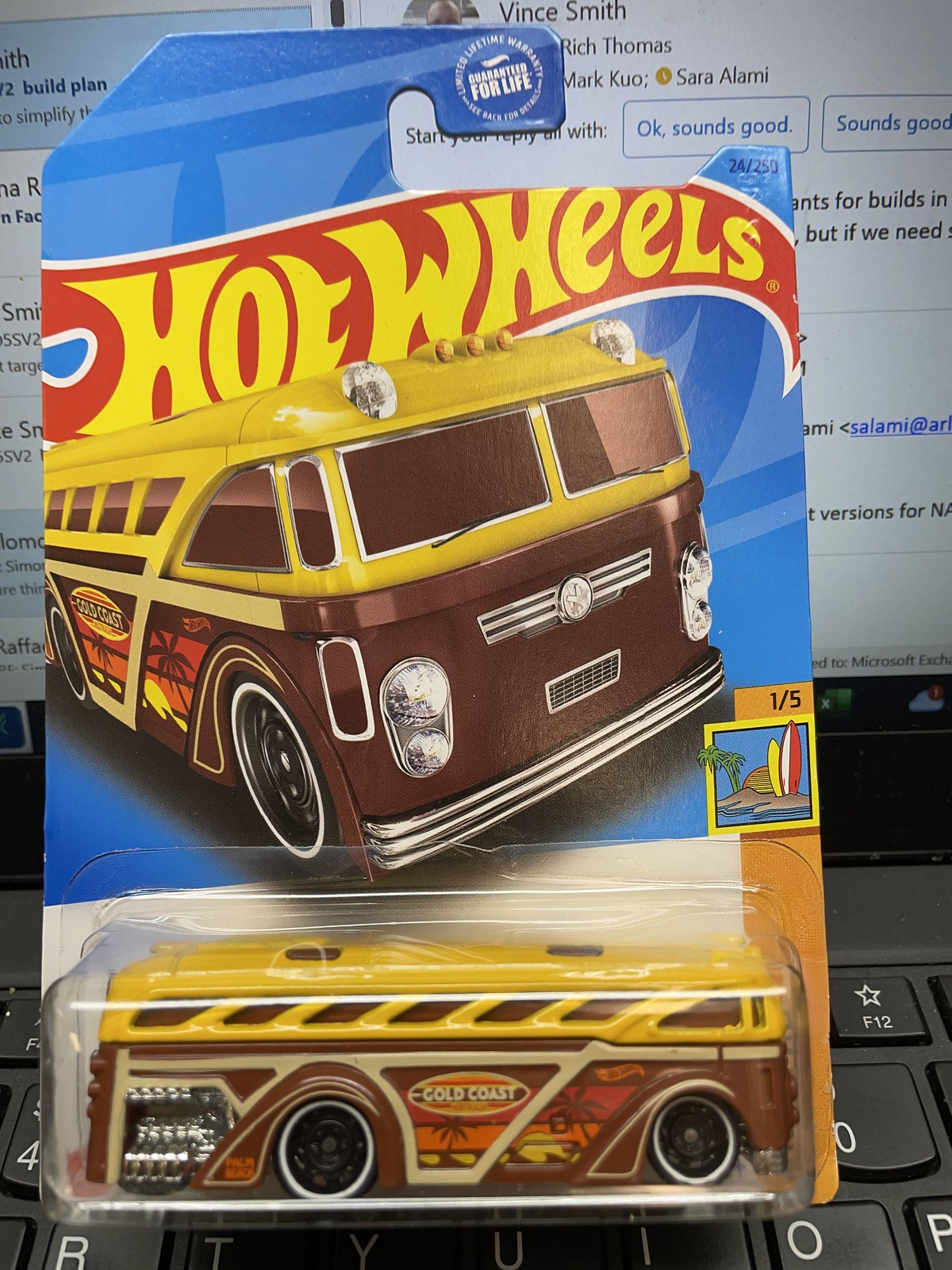A detailed close-up photograph features a well-preserved Hot Wheels toy still sealed in its original packaging. The toy is a Volkswagen-style bus, sporting a brown body with a contrasting yellow top. It rolls on black wheels accented with white wall tires. The packaging comprises a clear plastic bubble that showcases the toy, mounted on a colorful cardboard backing. This backing prominently displays a front view of the Volkswagen bus set against a blue background and is branded with the iconic Hot Wheels logo—a red flowing emblem containing the yellow text "Hot Wheels."

Above the toy, the backing card also mentions "Gold Coast," hinting at a beach vibe reminiscent of a 1960s van. A notation of "1 out of 5" suggests that this model is part of a limited series. The setting of the photograph indicates an indoor environment, implied by the open laptop in the background. The laptop screen reveals an email interface, giving context that the picture was likely taken while the person was engaged in emailing. The image, brimming with details, offers a nostalgic glimpse into classic toy collectibles juxtaposed with modern daily activities.